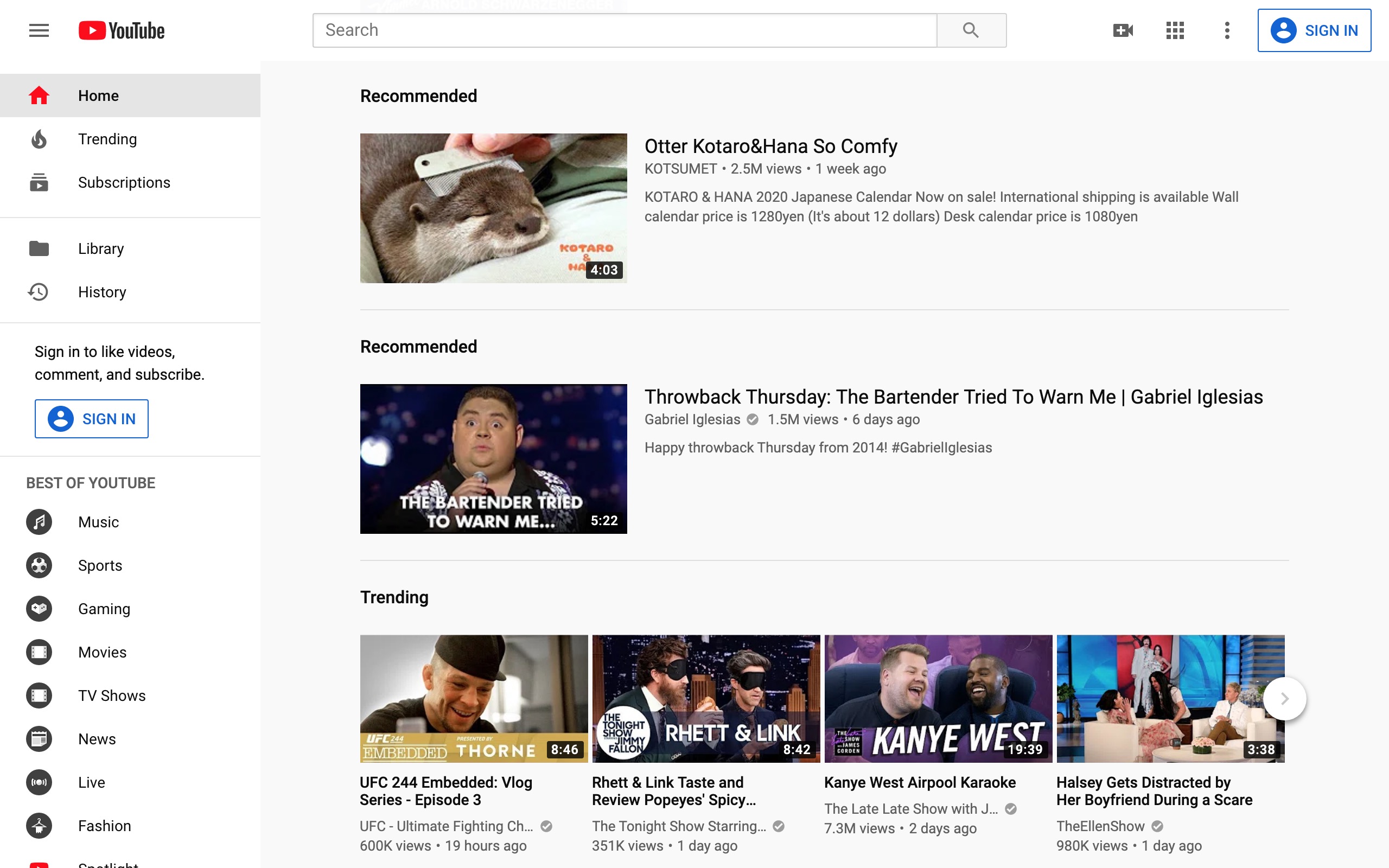This image captures a detailed view of the YouTube website interface. In the upper left-hand corner, the iconic YouTube logo stands prominently. To its right, a search bar invites users to find content across the platform. Directly below the logo, several navigational tabs are listed sequentially: Home, Trending, Subscriptions, Library, and History. There's also a prompt requesting users to sign in to like videos, comment, or subscribe, accompanied by a “Sign In” link.

Further down the interface under the header "Best of YouTube," various categories such as Music, Sports, Gaming, Movies, TV Shows, News, and Fashion are listed, though the full list extends beyond what can be viewed in this image.

Below the search bar, recommended videos for the day are displayed prominently. The first recommendation features a thumbnail image of a sea otter with the title "Otter Katoro and Hanna So Comfy." The description notes that the Katoro and Hanna 2020 Japanese calendar is now available for purchase, priced at 12.80 yen (approximately $12) for the wall calendar and 10.80 yen for the desk version.

The next recommendation appears to be a comedy clip from Gabriel Iglesias titled "Throwback Thursday: The Bartender Tried to Warn Me." The description celebrates Throwback Thursday with a mention of 2014 and hashtag Gabriel Iglesias.

This detailed view provides a comprehensive look into the various features and content offerings on YouTube’s homepage.